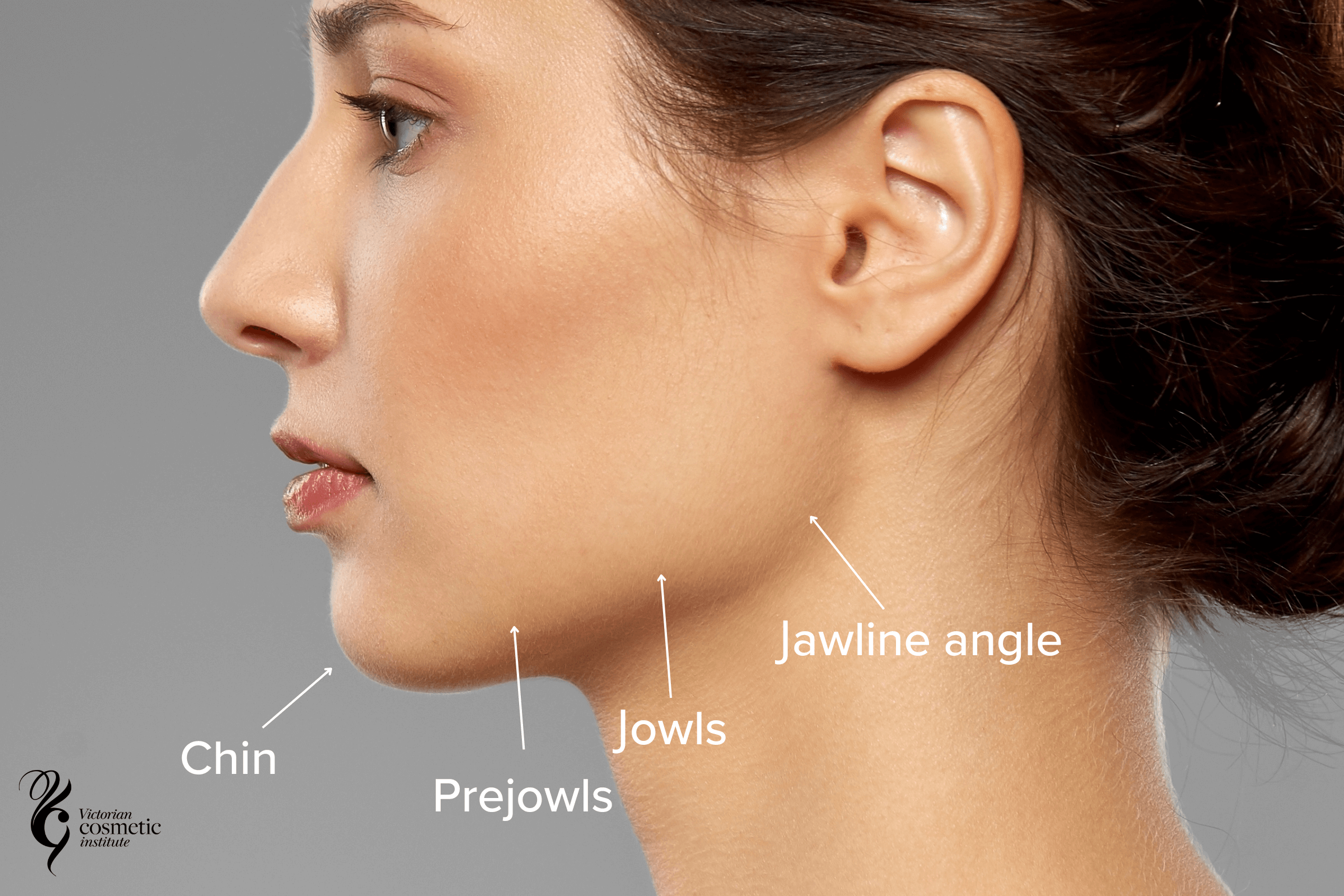The image depicts a Caucasian woman with olive-toned skin, shown in side profile looking to the left against a grey background. Her brown hair is up, likely in a ponytail or bun, although the exact style is unclear due to cropping. The focus is on the lower half of her face, illustrating her chin, pre-jowls, jowls, and jawline angle with arrows and labeled text. Her skin appears smooth and flawless; she has pink lips and piercing holes in her earlobes, though she is not wearing any jewelry. The image is cropped just above her eyebrows, showing only a part of her head and cutting off the top. In the bottom left corner, the Victorian Cosmetic Institute is mentioned in small text accompanied by a logo.